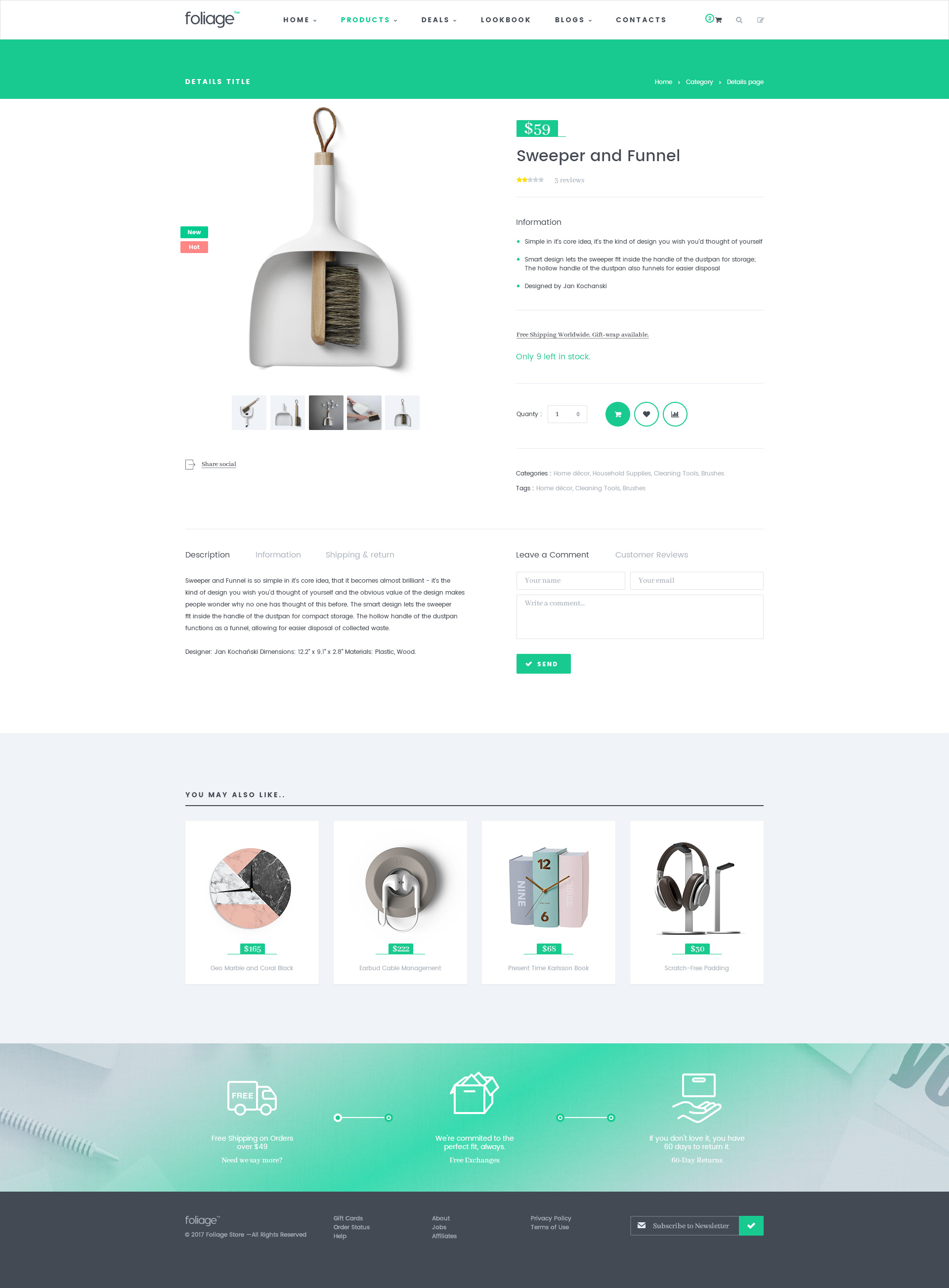The image depicts a detailed view of a commercial website, likely focused on home or cleaning products. At the top of the page, there is a prominent white banner featuring the company logo indicative of foliage, accompanied by a navigation bar with categories such as "Home," "Products," "Deals" (highlighted), "Blog," and "Contact." Icon links are positioned adjacent to these categories.

Beneath the main banner, a very light green section contains text (illegible from the image). The main content area below showcases a featured product—a hand broom neatly tucked inside a dustpan, with its handle upright. Directly underneath, there are five related images, possibly providing different views or variations of the dustpan and broom set.

To the right of these images, a product title "Sweeper in a Funnel" is displayed along with its ratings and a detailed description. Below this section, there are circular icons (their specifics are unclear) followed by a descriptive paragraph, a dividing line, and a comment section featuring a noticeable green submission button.

Further down, there is a gallery of four media images, each linked to various products, with associated text and green rectangular highlights underneath them - content is difficult to discern.

At the bottom, an icon of a truck symbolizes the shipping process, complemented by a black banner presenting additional information, possibly related to shipping or terms of service.